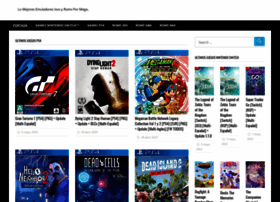The image displays an interface with a white background outlined in black, featuring a central search bar. Beside the search bar is a blue square containing a white magnifying glass icon, presumably indicating search functionality. Below the search bar, there are five movie icons arranged in a row.

The first icon is divided into two color blocks: the upper half is blue, and the lower half is red. The content of the icon pertains to movies, although details beyond the color scheme are not specified.

The second icon shows a man singing into an old-fashioned, silver, oval-shaped microphone, suggesting a musical or performance-related theme.

The third icon features a cartoon character in motion, depicted as running, hinting at an animated or action-oriented movie.

The fourth icon portrays a man in a suit with a sneaky demeanor, potentially indicative of a spy or thriller film.

The fifth icon features a man walking outdoors at night. The context suggests the presence of "dead cells," which could imply a horror or sci-fi movie theme involving danger or infection.